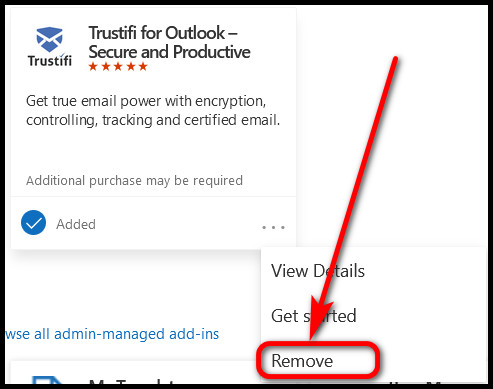In the provided image of a webpage section, the main visual centers around an icon located at the upper-left. This icon, shaped like a shield, incorporates a blue envelope design, symbolizing security and communication. Directly below the icon, the text "Trustify" is written in black. Adjacent to the icon, the heading reads "Trustify for Outlook, Secure and Productive" with "Secure" emphasized by five red stars underneath. 

Below the stars, additional text in black promotes the software's features: "Get True Email Power with Encryption, Controlling, Tracking and Certified Email." A disclaimer stating "Additional Purchase May Be Required" is positioned beneath this promotional text. Further down, a white checkmark enclosed in a blue circle is placed next to an unspecified word, indicating a likely list item or feature.

In the lower right corner, there is a red oval encircling the word "Remove," with a red arrow pointing towards it, highlighting a call-to-action or interactive element on the page.